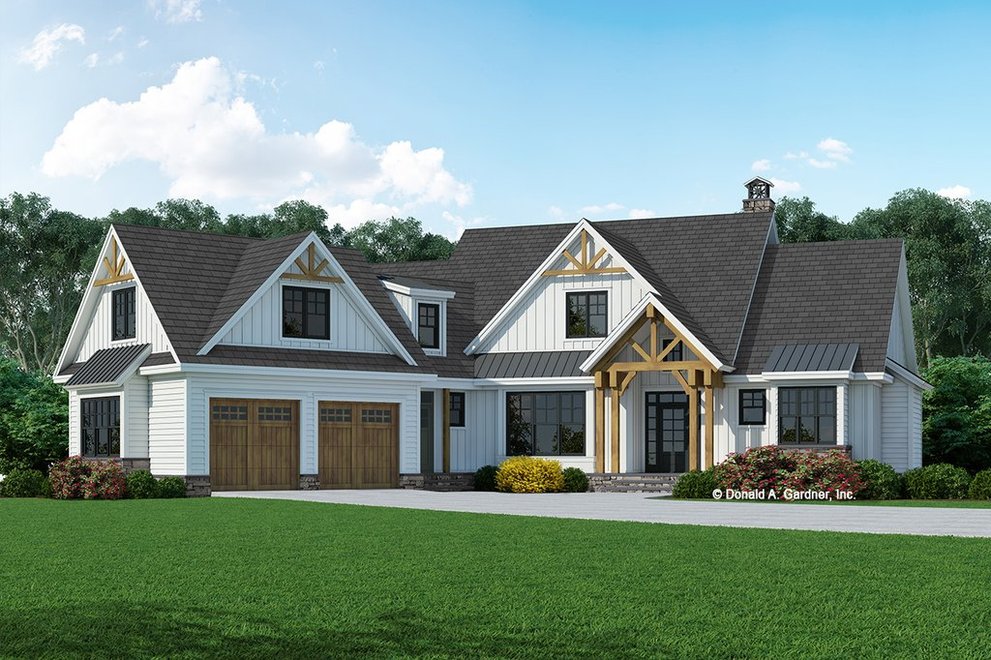The image captures a pristine, two-story gabled house featuring an impeccably manicured lawn of short, verdant grass. The house is characterized by a dark gray or black roof with wide triangular fronts and dormer-style windows. The second floor showcases four prominent windows set beneath the triangular sections of the roof, all framed against the house's stark white walls. At ground level, the structure includes two garage doors, both brown, with a long driveway extending from the left garage door across the front of the house. A wooden-framed entrance door is located on the right side of the house. The overall appearance of the scene is extraordinarily flawless, almost too perfect, giving it an unsettling, possibly computer-generated aura. A text reading "Donald A. Gardner Inc." is visible to the right of the scene, indicating perhaps the designer of this impeccable, picture-perfect home.